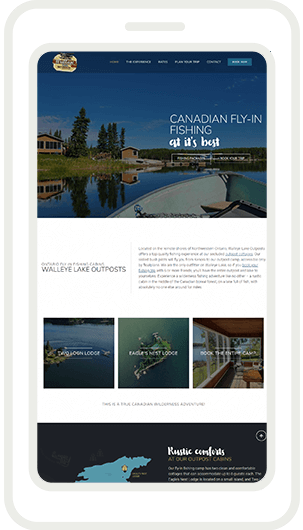This image is a digitally superimposed advertisement resembling a webpage displayed on an elongated, portrait-oriented cell phone screen. The screen simulation features a tall, rectangular gray border with rounded edges, mimicking the frame of a mobile device. Inside this border, a slightly thicker gray outline frames the webpage, creating a contrast with the white space in between.

The webpage itself has a vibrant header strip comprising a yellow circular logo with a red banner to the left, set against a blue horizontal background. The word "Home" stands out in yellow, accompanied by several smaller, unreadable white text items. A long, light blue rectangular button with white text is also present but illegible.

Beneath the header, the main image showcases a picturesque scene featuring a sky, grassy banks, trees, cabins, and a lake, captured from the vantage point of a boat. Overlaid on this image is the bold statement: "Canadian Fly-In Fishing at its Best."

Further down, on the left, the words "Walleye Lake Outpost" are displayed above a descriptive paragraph on the right. The page concludes with three thumbnail images, each presumably representing different lodges available for accommodation. These thumbnails appear clickable, likely leading to more detailed images or information about each lodge.